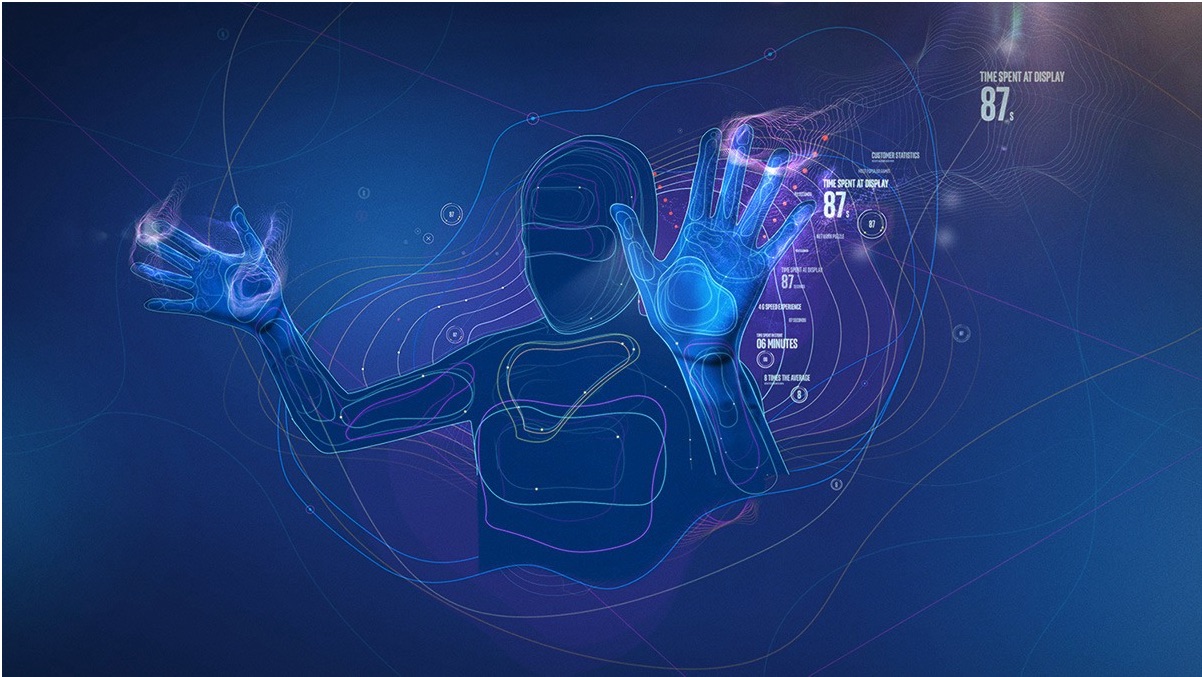The image is a formally aligned, rectangular, computer-generated design primarily featuring different shades of blue and purple. The background is a dark blue, resembling the night sky, with numerous small white bubbles floating around. At the center of the image is an outline of a person, depicted from the head to the stomach, with their hands outstretched and palms facing forward. The hands have highlights that give them a three-dimensional appearance, while the rest of the body appears flat due to the lack of highlights.

Various warped and thinly drawn lines radiate from the person, forming a circular pattern. These lines, in colors such as white, purple, blue, green, and orange, create spiral shapes behind the figure, contributing to the sense of movement and energy. More lines trace different shapes on the person's chest, including curved rectangles and triangles in blue, green, or purple, adding to the intricate detail of the image.

Additionally, there is text and numbers present in the image, particularly noticeable in the upper right corner, where it reads "time spent at display" followed by "87s." This text and other details, along with the structured and dynamic use of lines and colors, suggest that the image might be part of a video game interface or a digital artwork.